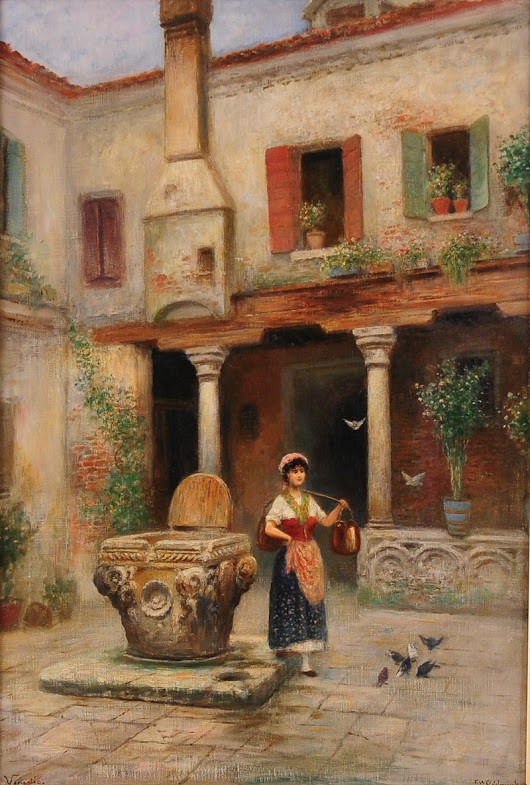This painting, likely European in origin, depicts a serene and colorful rural scene featuring a woman standing beside an archaic well adorned with circular and intricate designs. The well has a wooden lid that appears to be functional, opening and closing as needed. The woman, clad in traditional, old European attire—a dark blue dress with white and red accents and a hat—carries two brass containers on a yoke over her shoulder, presumably filled with water recently drawn from the well.

She stands on a brick surface, surrounded by a picturesque environment that includes six birds on the ground, with a couple more flying nearby. The backdrop showcases a charming, sepia-toned house with a combination of exposed brick and peeling cement. There are potted plants and vibrant flowers in the open and closed shutters, some of which are a brick red and others a teal green. Ivy climbs the walls of the house, adding to the antiquated beauty of the scene. The presence of windows on the house with plants in them, along with the lush greenery surrounding the area, creates a vivid and captivating portrayal of a tranquil, rustic moment frozen in time.